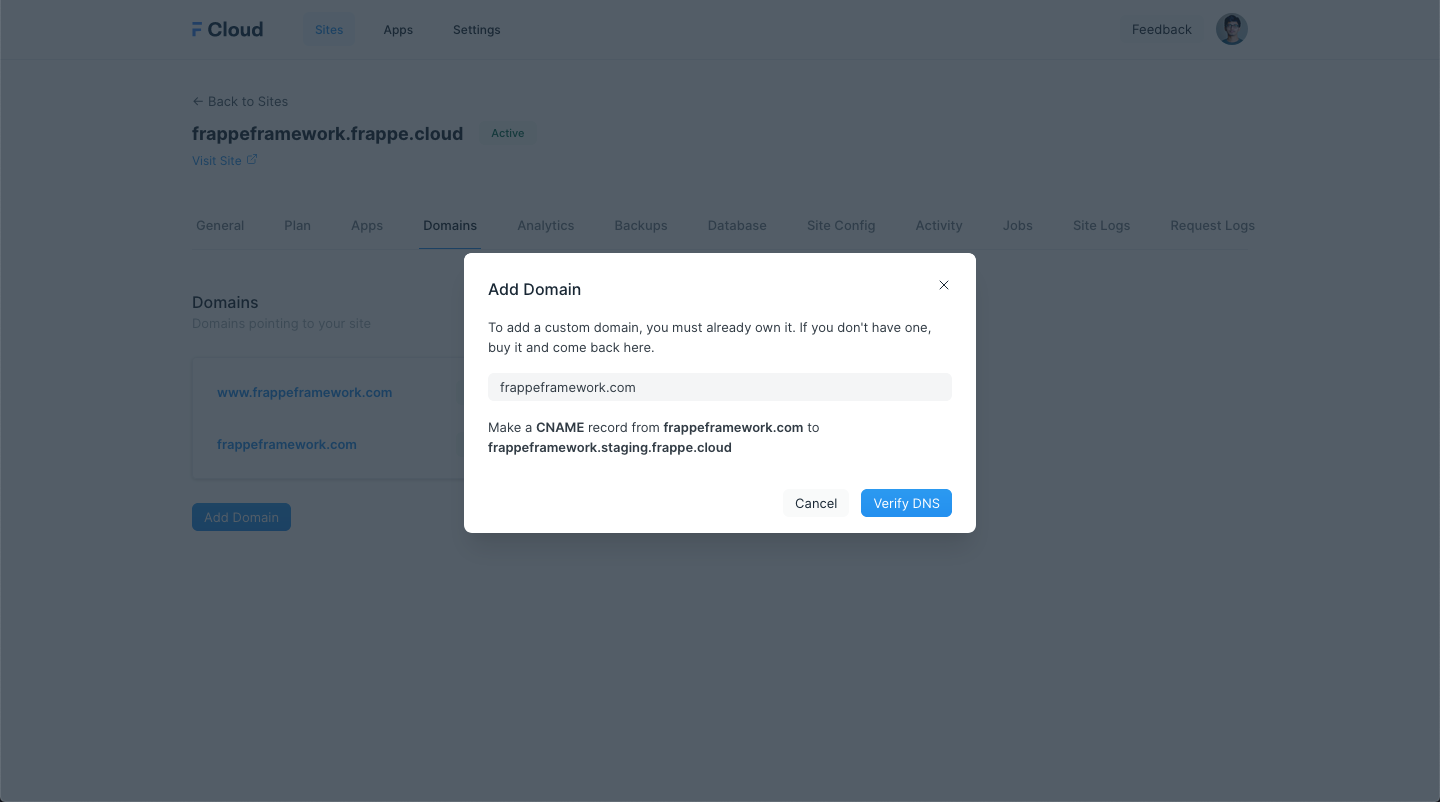The image is a screenshot from a web-based management interface for the FRAP cloud framework. In the background, there is a navigation panel displaying various sections of the platform, such as sites, apps, settings, FRAP framework, and cloud services. The active tab is the 'Sites' section, which offers options like general settings, plan details, apps management, analytics, backups, and database handling. Additionally, there are multiple instances of the 'Domains' section listed, emphasizing its importance. 

The main content area provides specific instructions for adding a custom domain to your site hosted on FRAP.cloud. It guides the user through the necessary steps: First, they are prompted to ensure they already own the domain name they wish to add. If they don't, they are advised to purchase one and then return to the interface. 

Next, the user is instructed to create a CNAME record, pointing from their domain (e.g., 'www.frapwork.frapframework.com') to 'frapframework.staging.frap.cloud'. The interface also includes options to cancel the operation or to verify the DNS settings once the CNAME record has been properly configured. 

The foreground prominently features a button labeled “Add Domain” which is the user action point for initiating the domain addition process.